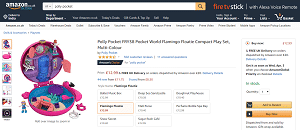The image depicts a typical product page on Amazon.com, featuring a children's toy targeted at girls. The interface showcases the customary Amazon layout, with the search bar at the top. To the left, there's the Amazon logo, while the top-left corner displays the Amazon Prime badge. Adjacent to this, there's a clickable Fire TV Stick advertisement. The product section is quite detailed: on the left side, there’s a photo carousel offering various views of the toy. The right side prominently displays the product's price in red font and availability in green font, indicating that the item is in stock. Users can choose to add the item to their cart or buy it immediately through the "Add to Cart" and "Buy Now" buttons. Above these options, there's a field to select the desired quantity. Beneath the search bar, several category links are available for further navigation. Additionally, the cart icon at the top-right corner suggests that there are items currently in the cart, though the exact number is unclear. The entire page is set against a clean white background, maintaining the familiar and user-friendly Amazon aesthetic.